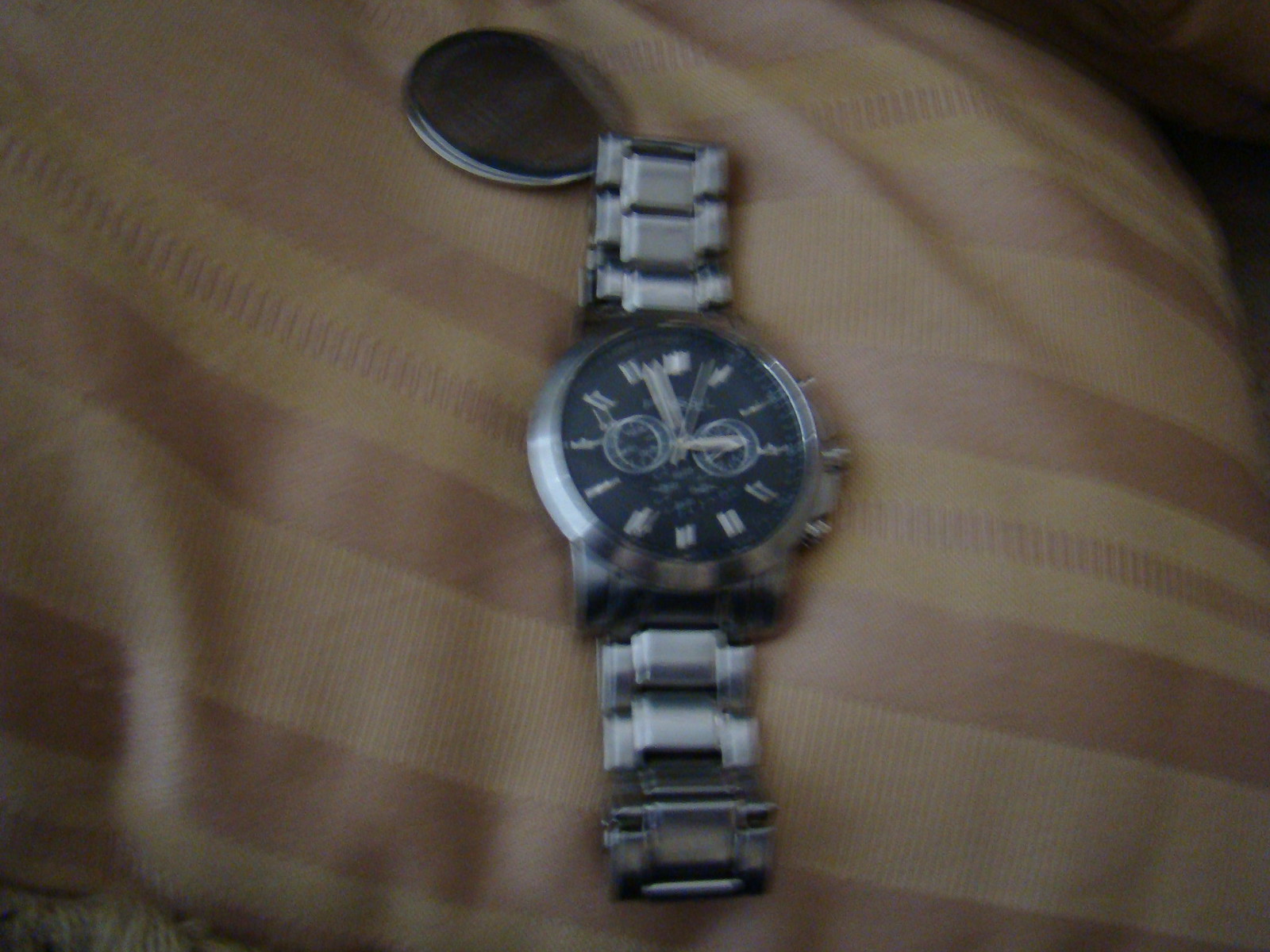A men’s silver watch with black accents rests on a surface that appears to be a striped fabric, possibly a pillow, blanket, or shirt. The fabric features alternating stripes of tan and dark brown, creating a textured appearance. The watch is facing up, but the image is blurry, suggesting the camera focused more on the fabric than on the watch itself. The back of the watch, with its silver plate, is positioned prominently in the image. The watch face includes multiple interfaces, likely displaying military time, seconds, and the date.